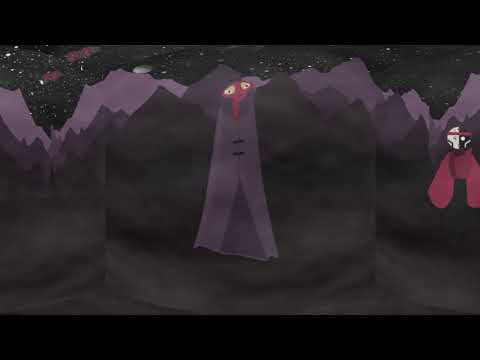The image portrays a dim, dark-themed scene, reminiscent of a child's drawing or an abstract artwork, dominated by hues of black, gray, and dark blue. The foreground features jagged mountains of varying heights and colors, notably black and dark grayish-purple, which run horizontally. The sky above is entirely black, speckled with small white dots resembling stars. In the center of the composition, a figure with a red face and neck, large white eyes, and draped in a dark gray cape stands prominently; this character appears two-dimensional with an animated feel. To the right, another figure is visible, characterized by a black and white circular head, wearing an outfit with a red poofy sleeve, evoking a yin-yang motif. The scene evokes an alien landscape beneath a starry night sky, with the central figure popping out amidst the spiky, mountainous terrain.